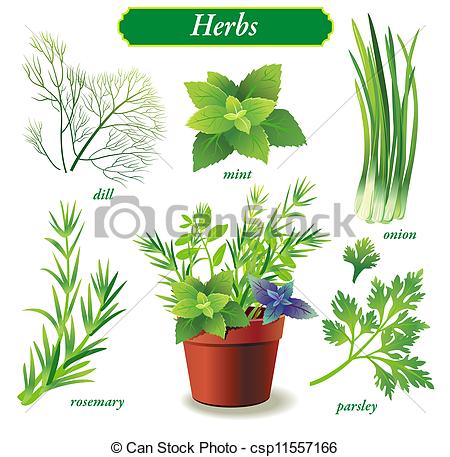This is a detailed, rectangular illustration of various herbs arranged around a central potted plant with blue flowers. At the top of the image, a green banner with white text reads "Herbs." Surrounding the pot, which is centrally positioned at the bottom middle, are multiple herb illustrations, each labeled with green text: to the left of the pot is rosemary, and to the right is parsley. Above the pot, from left to right, are illustrations of dill, mint, and onion, each with their names beneath them. A camera icon with the word "Genstock" is situated above the pot, while at the bottom, the image includes a copyright mark and text: "© CanStockPhoto-CSP11557166." The colors predominantly feature shades of green from the herbs, contrasting with the red pot housing the blue-flowered plant, creating a vibrant and informative depiction of various culinary herbs.